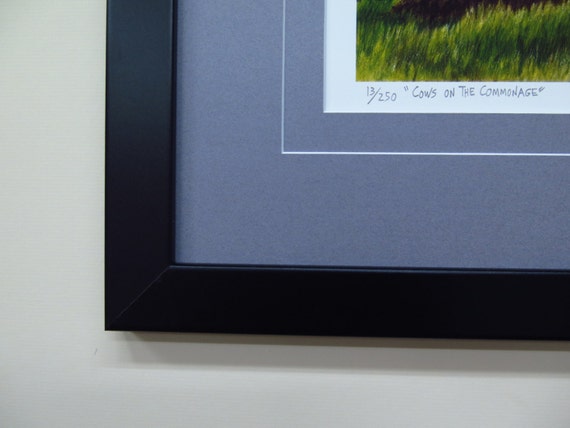The image is a close-up photograph of the bottom left corner of a black picture frame. The frame surrounds a light gray background with a thin white line slightly towards the center, both vertically and horizontally. This white line encloses the main artwork area, where green and yellow hues suggest the presence of grass. The canvas inside the frame is white and has a printed edition number and title along the bottom edge, reading "13/250" with the title "Cows on the Common Edge" quoted in black lettering. The frame is mounted on an off-white or grayish-white wall, casting a subtle shadow beneath it. The colors in the image include black, white, green, gray, and hints of yellow, creating a neutral and earthy palette.